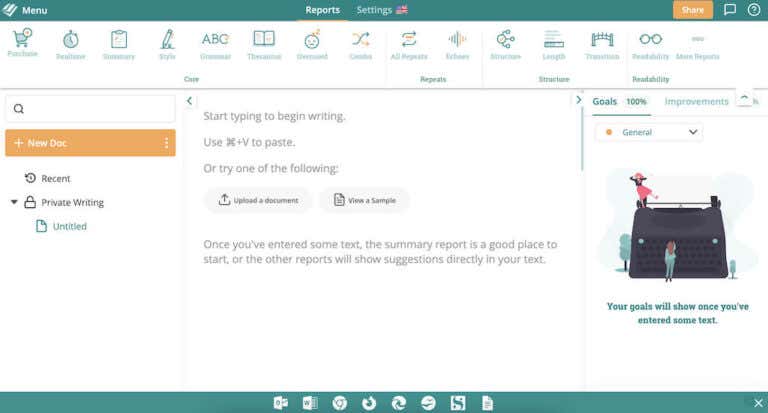Screenshot of a website page featuring a content management interface. The top section of the page is adorned with a winter-green header. On the far left of the header, there is a "Menu" option. Centered within the header are tabs labeled "Reports" and "Settings" alongside an indiscernible flag icon. The "Reports" tab is currently active. On the far right of the header, there are icons for sharing, commenting, and help functionalities.

Beneath the header, the background transitions to white. This section features various icons arranged horizontally that provide functionalities such as "Purchases" and "Translate." 

On the left-hand side, the user interface includes an orange-highlighted "New Doc" option, followed by various sections like "Recent," "Private Writing," and "Untitled." 

At the center of the page, there is a large, prominently white space with instructions to "Start typing to begin writing." It also offers options to paste text using "Ctrl+V," upload a document, or view a sample. Additional guidance suggests that the "Summary Report" is a good starting point once text has been entered.

To the right side of the page, there is a goal tracker displaying progress toward 100% completion and improvements. Below it, a drop-down tab labeled "General" can be expanded. Further down, a graphical representation indicates that goals will be displayed once some text has been entered.